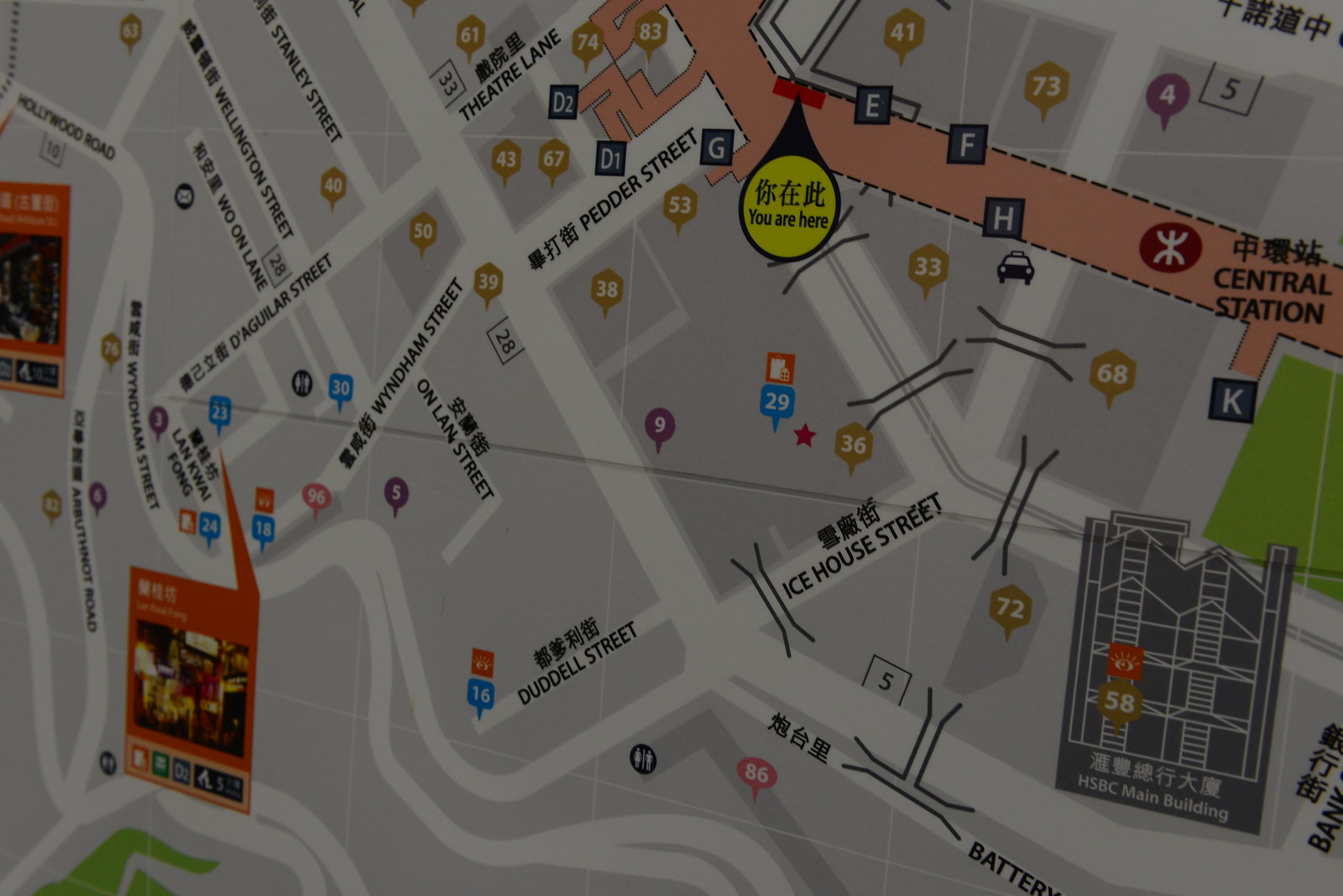This image is a detailed map of a city, possibly showcasing a bus stop or central locations within the city. The map is primarily gray with white strips depicting roads and pathways. In the upper portion, there's a prominent pathway colored in peach, suggesting a significant route through the city. Streets such as Wyndham Street, D'Aguilar Street, Icehouse Street, Pedder Street, Theater Lane, Wellington Street, Stanley Street, Hollywood Road, and more are labeled in both English and an Asian language.

Near the top of the peach-colored pathway, a yellow circle with Asian writing and the words "You Are Here" in black, accompanied by a black pointing arrow, marks a specific location. This yellow circle is connected to a smaller red rectangle. Central Station is noted towards the middle right of the map, accompanied by a letter "K" and more Asian text. Various points of interest are marked with color-coded circles and squares, including a number 58 indicating the HSBC Main Building.

Additional features include numerous letters such as D1, D2, E, F, and H spread across the upper part of the map, blue numbers, red bars, and car logos. The map also contains several icons and notations, employing a style indicative of color illustration and graphic design. The orientation of the image is landscape, giving a bird's-eye view of the area.